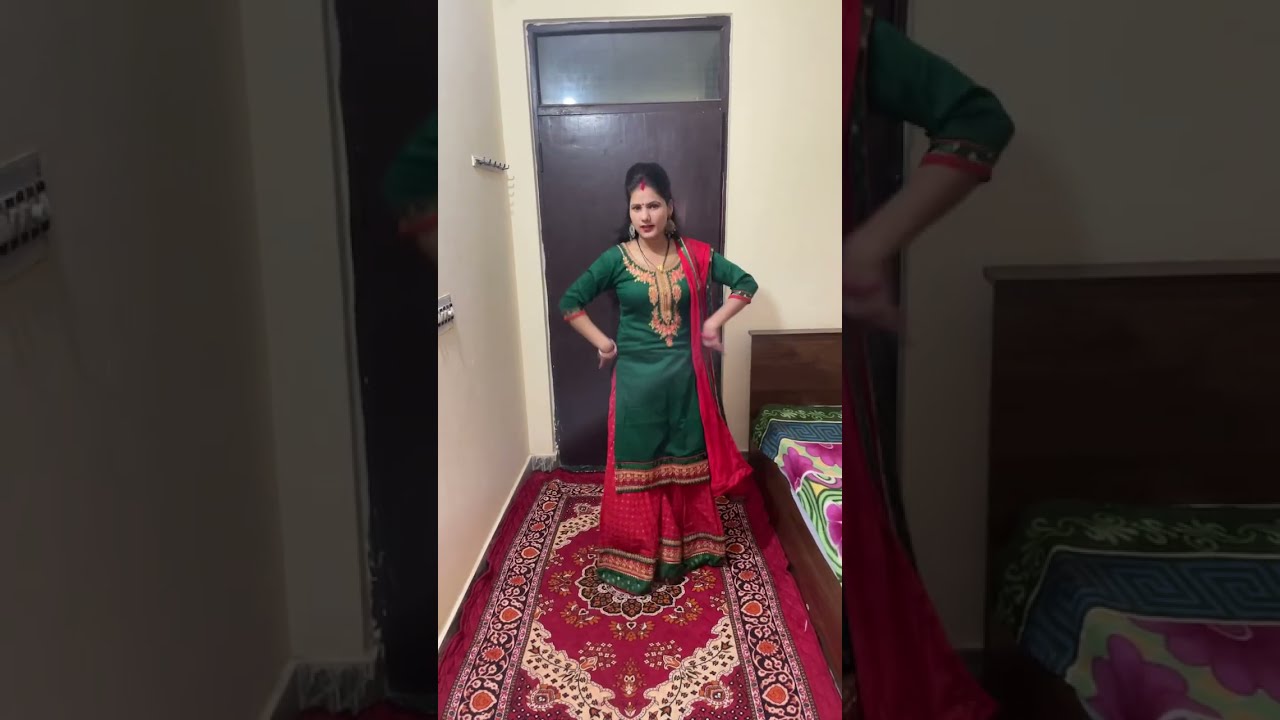The photograph features an Indian woman elegantly dressed in a colorful traditional outfit. Her ensemble includes a red skirt and a green top adorned with intricate gold embroidery. Draped over her left shoulder is a red silk scarf that flows down her front, enhancing the decorative attire. The woman, with her black hair neatly set, stands confidently on a richly patterned red rug, with both hands firmly placed on her hips. Her accessories include gold earrings and bracelets, and a red dot adorns her forehead, adding to her traditional look.

She stands in front of a brown door, with a bed to her right and a wall to her left. The image is a horizontal rectangle divided into three parts: the central part is a clear and well-lit shot of the woman, while the sections on the left and right are darker, blurred close-ups of the same image. These blurred sections frame the sharp, detailed center, highlighting the vividness of her attire and the room's decor, including the door, walls, and bed. The overall color palette of the image includes red, green, gold, dark brown, white, tan, pink, and yellow, creating a vibrant and culturally rich scene.